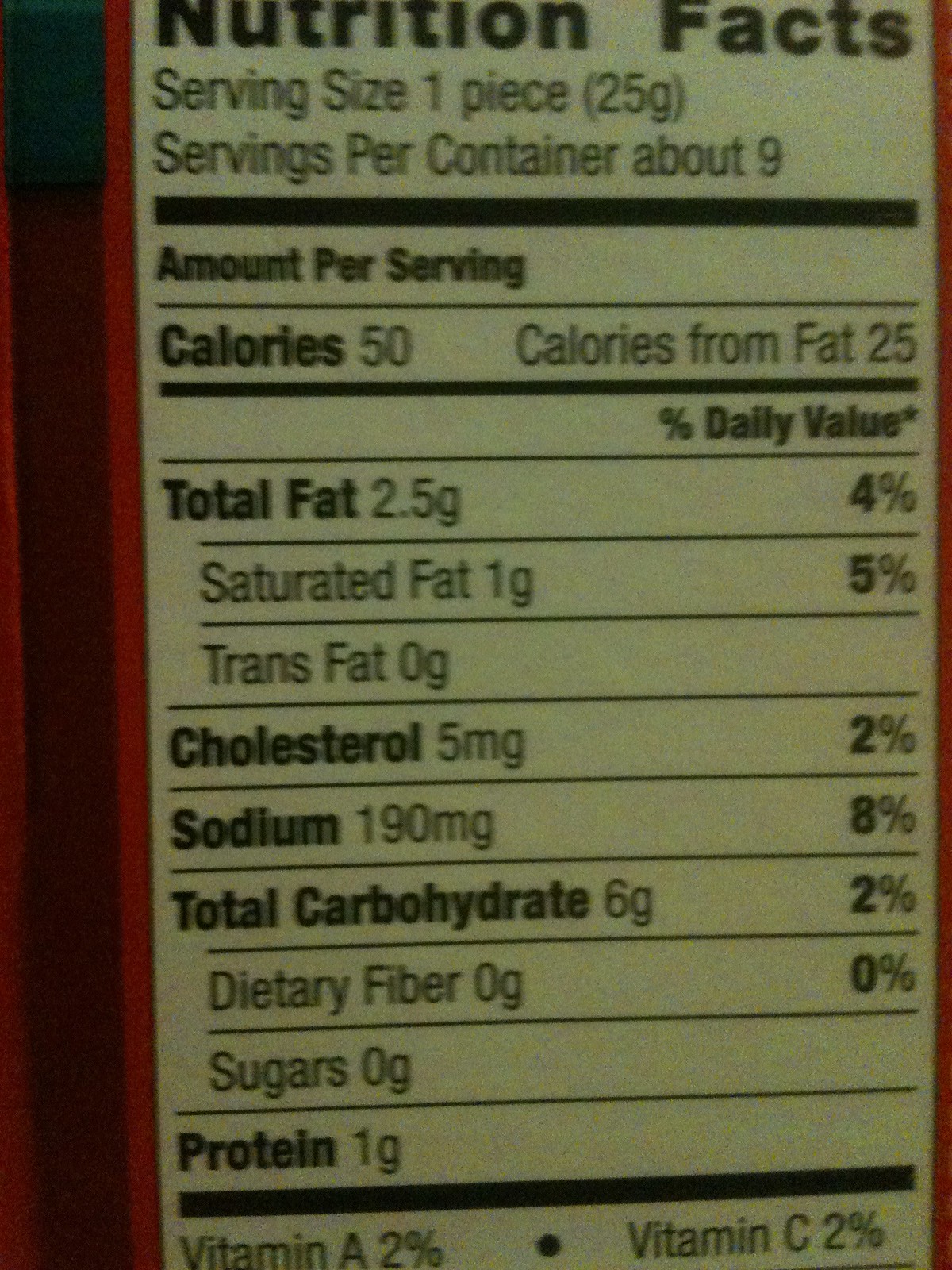The image captures a close-up view of a nutrition facts label, though it is somewhat cut off at the top and bottom. The quality of the image is slightly grainy, and the label is framed by a light red inner border and a darker burgundy outer border. Despite the cut-off portions, the label provides detailed nutritional information.

**Nutrition Facts:**
- **Serving Size:** 1 piece (25 grams)
- **Servings Per Container:** About 9
- **Amount Per Serving:**
  - **Calories:** 50
  - **Calories from Fat:** 25
  - **Total Fat:** 2.5 grams (Saturated Fat: 1 gram, Trans Fat: 0 grams)
  - **Cholesterol:** 5 milligrams
  - **Sodium:** 190 milligrams
  - **Total Carbohydrates:** 6 grams (Dietary Fiber: 0 grams, Sugars: 0 grams)
  - **Protein:** 1 gram
  - **Vitamin A:** 2%
  - **Vitamin C:** 2%

The absence of sugar, combined with the general content information, makes it difficult to pinpoint exactly what this product is. The label's clarity is compromised by the grainy quality and partial cutoff of the image, further adding to the curiosity about the nature of the item.